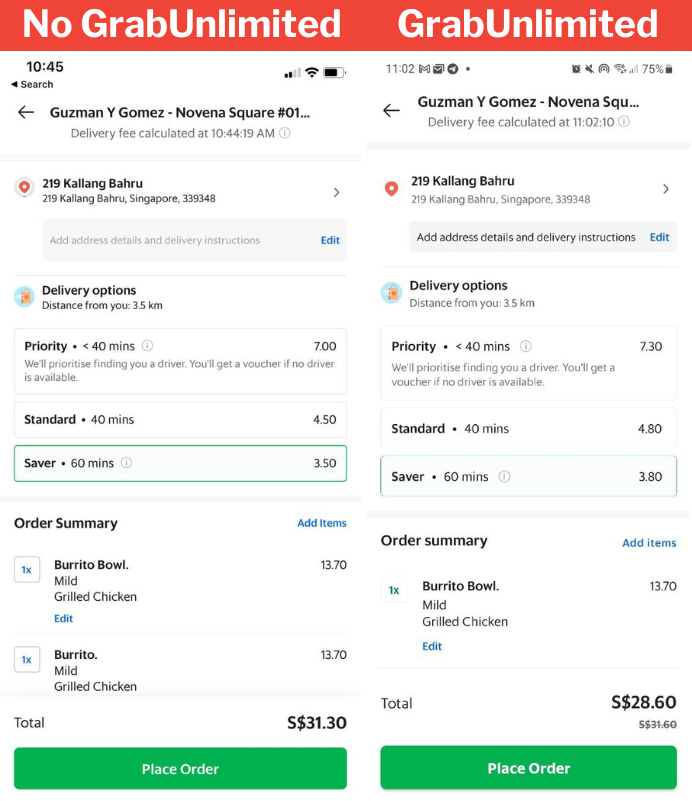The image displays two smartphone screenshots placed side by side, each showcasing an order from a food delivery app. 

At the top, an orange bar runs horizontally across both screenshots, displaying different text:  
- On the left, it reads "no grab unlimited."
- On the right, it says "grab unlimited."

Each screenshot includes common smartphone iconography at the top corners and a "Place Order" button at the bottom. 

### Left Screenshot:
- **Total:** $31.30 
- **Header Details:** The name of the restaurant, "Guzman y Gomez Novena Square," and the address "219 Calang, Peru."
- **Content:** Delivery options and an order summary are visible.

### Right Screenshot:
- **Total after savings:** $28.60 
- **Savings Indicated:** "Saved $31.60," implying that the original price was $31.60.
- **Header Details:** Same as the left screenshot, displaying "Guzman y Gomez Novena Square" and "219 Calang, Peru."
- **Content:** Similar delivery options and order summary present.

Both screenshots offer a comparison in pricing and options between a standard order and a "grab unlimited" membership, showcasing the discount achieved with the membership.